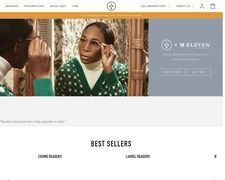The image depicts a sophisticated woman gazing at herself in a mirror, showcasing her stylish ensemble. She wears a green V-neck sweater layered over a cream-colored turtleneck. An elegant black woman, her appearance is thoughtfully accessorized with glasses held delicately by her right hand. Her hair is neatly pulled back, emphasizing her refined look.

Behind her, a set of cream-colored curtains with green accents frames the scene, adding a touch of elegant ambiance. The image likely serves as an advertisement for eyewear, as indicated by the "bestsellers" label below the mirror depiction, featuring two popular styles.

Adjacent to the right side, the name "Evelyn" appears, accompanied by a subtle gray logo of the company to the left. Beneath the advertisement, a gray bar invites interaction, suggesting that viewers can click the names of the bestsellers for more details. This image seems to be part of an online shopping site, complete with icons at the top to assist potential buyers.